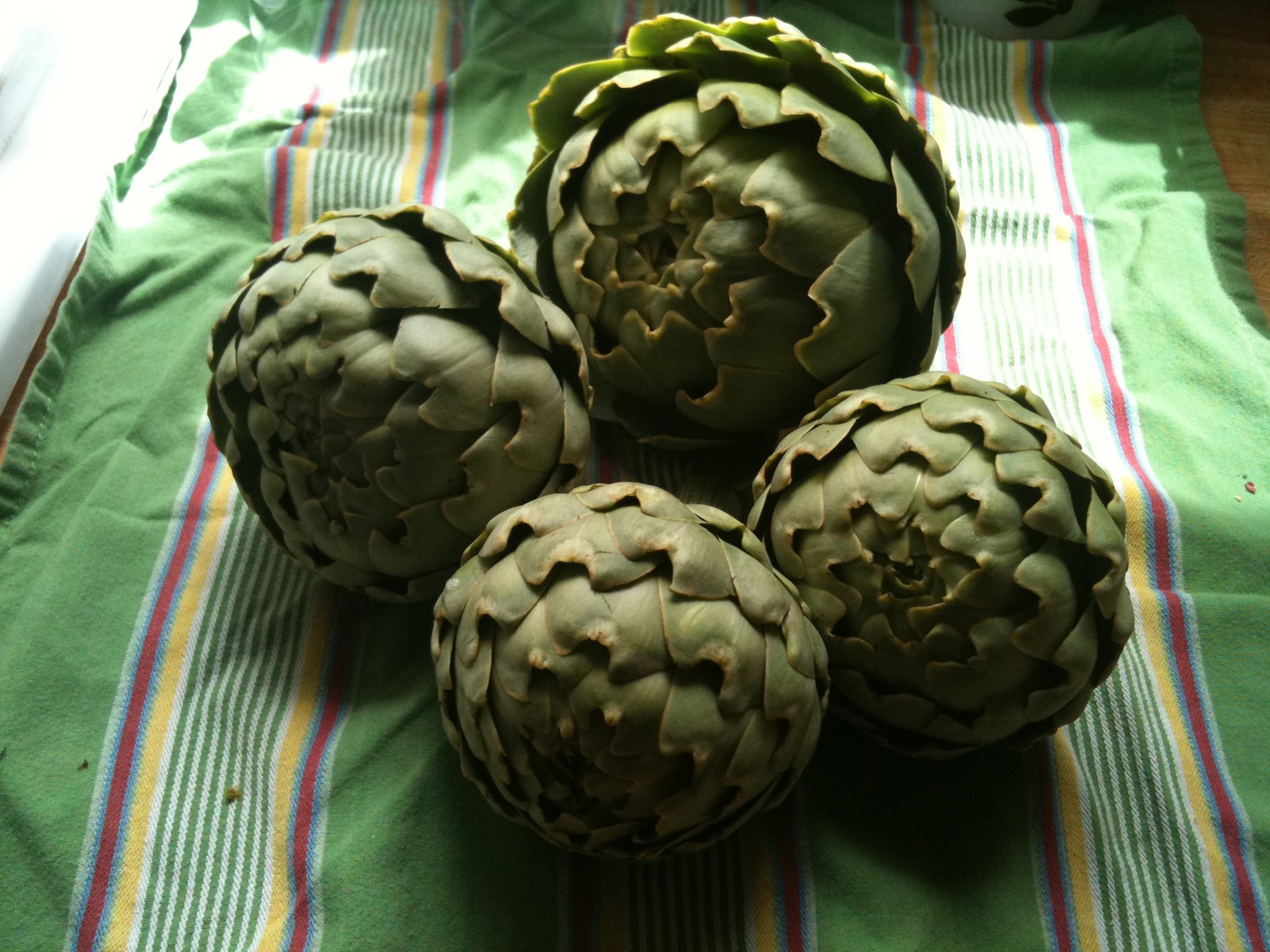In this photograph, we're presented with a close-up view of four green artichokes arranged on a brown wooden table. The artichokes are resting on a green cloth that features colorful vertical stripes in red, white, yellow, and hints of blue. The stripes run down the center of the cloth, adding a vibrant contrast to the earthy tones. The artichokes themselves are positioned with their tops facing the viewer, revealing the overlapping leaves that give them a textured, scale-like appearance. The four artichokes vary in size: the largest one is in the upper right, followed by a slightly smaller one in the upper left, while the two at the bottom are the smallest and similar in size. Soft light filters in from what appears to be a nearby window, giving the scene a natural, indoor ambiance.